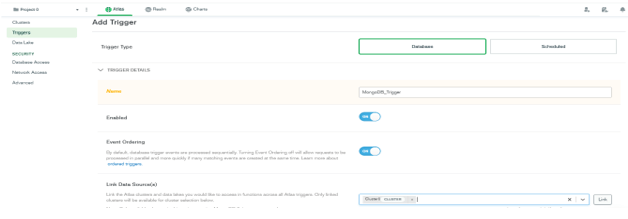The image depicts a webpage with a navigation menu on the left side, although the resolution is quite poor, making it difficult to read the specifics. The navigation menu appears to list several items, starting with what seems to read "proposal zero" followed by some sort of dropdown or pull-down menu. Below that, there are several other items; one of them is titled "triggers", highlighted in green, indicating it is the current selection.

In the main content area, the page is focused on an "add trigger" section. This section includes options such as "add trigger" at the top, followed by what looks like "trigger type" and potentially "trigger contents" with a dropdown. There is text written in yellow below these fields. Additionally, there are options for "enable" and "event ordering," both associated with toggles that are turned on and displayed in blue. Underneath, there is some more text, mostly in black and blue, though it is largely unreadable due to the low resolution. The text might potentially include a date field, but this is not clear.